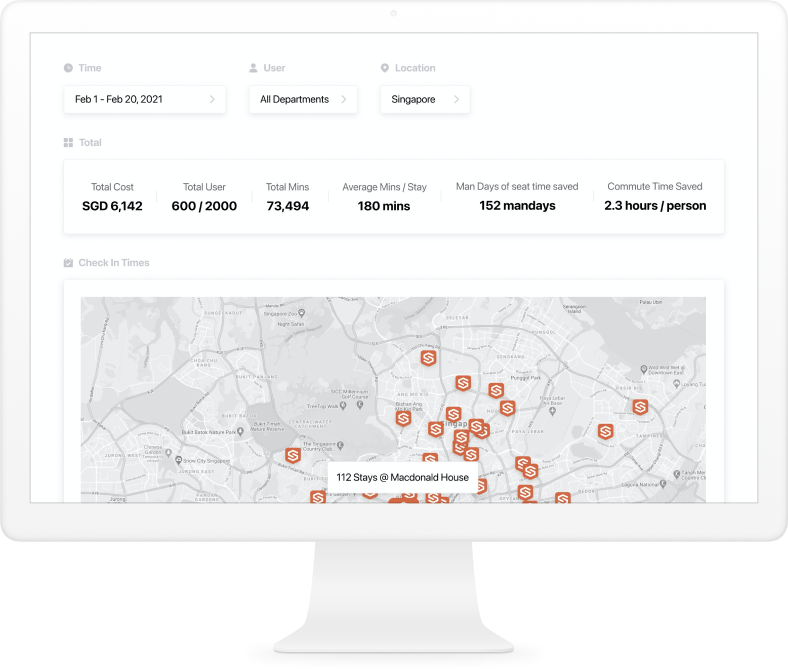This image captures a snapshot of a computer screen displaying a detailed report related to time usage and related statistics for all departments within a location in Singapore, covering the period from February 1st to February 20th, 2021. 

Key metrics shown on the screen include:

- **Total Cost:** SGD 6,142
- **Total Users Engaged:** 600 out of 2000 
- **Total Minutes:** 73,494 minutes
- **Average Minutes per Session/Stay:** 180 minutes
- **Man-Days of Seat Time Saved:** 152
- **Commute Time Saved:** 2.3 hours per person

Additionally, the report highlights check-in times and includes a map adorned with red triangles containing dollar signs, which represent various McDonald’s house locations in the area. Notably, the data indicates there have been 112 stays at McDonald's house.

The screen is shown on an all-in-one white PC with a sleek white stand, contributing to a modern and clean look. The interactive map component of the display allows users to click on the icons for further detailed information regarding check-in schedules and specific locations.